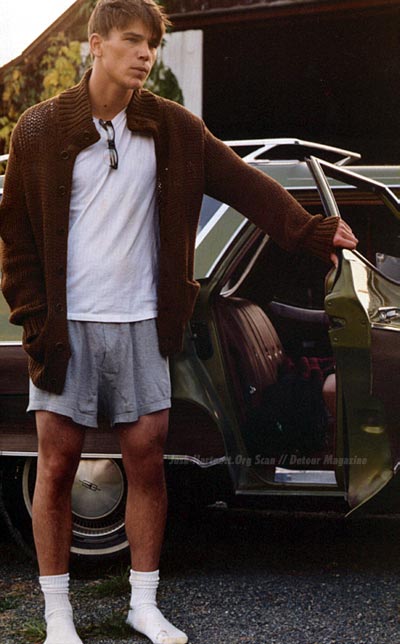The image is a detailed photograph, likely a screen grab from a movie, featuring actor Josh Hartnett. He stands solemnly with a neutral expression, positioned slightly to the left side while holding open the door of a green station wagon with brown seats and wood grain panels. Josh is casually dressed, donning a brown knit sweater jacket over a white undershirt, tucked into gray shorts or gym pants, complemented by white athletic socks. His short brown hair is unstyled, and he has sunglasses clipped to his undershirt. The scene is set on a gray asphalt driveway, with a modest house in the background and a small green-leafed tree about 15 feet tall in the distance. The sky is partially visible above.